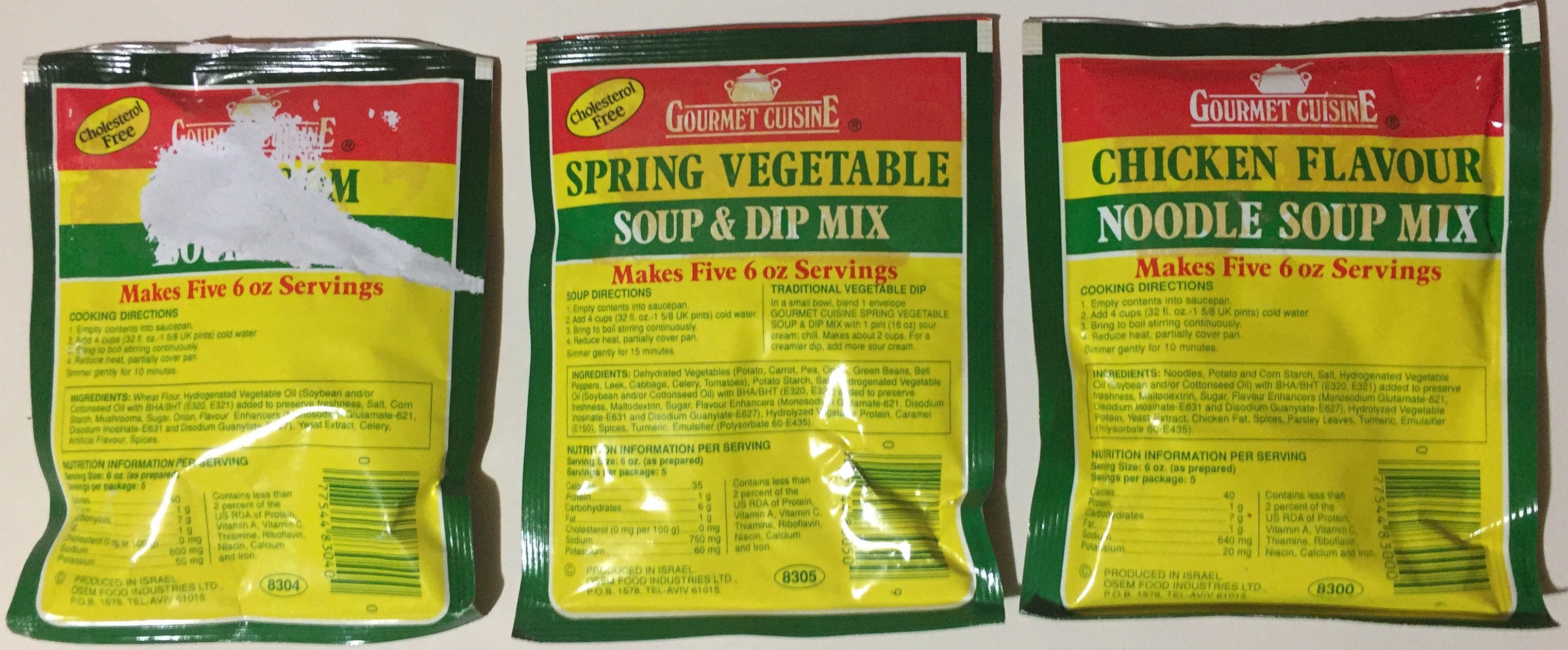This is a detailed photograph showcasing three packets of soup and dip mix, arranged neatly in a horizontal row against a light gray background. Each packet casts a subtle shadow on the surface below, adding depth to the image. The packets are identical in brand and packaging, though they present different flavors. The design features a red banner at the top, followed by a yellow stripe, then a green stripe, with the remainder of the package in yellow. The first packet has noticeable damage where part of the packaging, including the flavor label, has been scratched off, leaving its flavor unknown. The second packet is labeled as Spring Vegetable Soup and Dip Mix, while the third packet displays Chicken Flavor Noodle Soup Mix. All three packages remain sealed and untouched, indicating they are full and unopened.